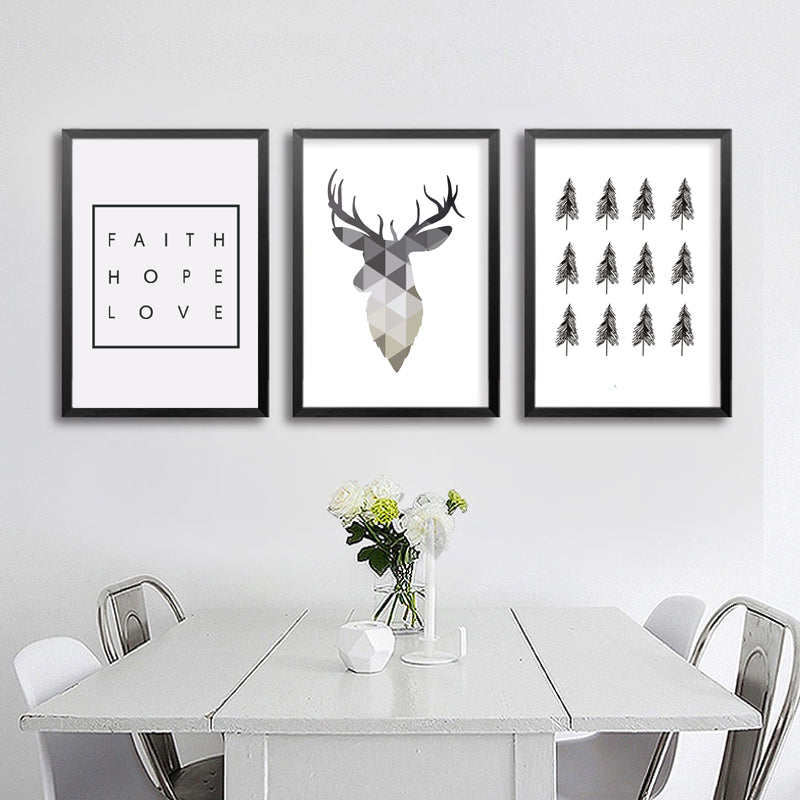In a cozy dining area with a white wall, three striking black-framed prints hang above a reflective white wooden table. The first print, situated to the left, features the words "Faith, Hope, Love" inside a black square. The middle print showcases a geometric buck, its body composed of intricate triangular patterns in shades of gray, black, and white, with solid-colored antlers. The third print displays a neat arrangement of twelve evergreen trees, set in three rows of four. Beneath these prints, the table is surrounded by four chairs—two sleek white plastic ones at the lower left and upper right, and two metal barn-style chairs with thin backs at the upper left and lower right. On the table, a clear vase holds a bouquet of white and yellow flowers, accompanied by an ultra-thin white candle and a geometric, stemless apple-like object, adding modern and natural touches to the space.